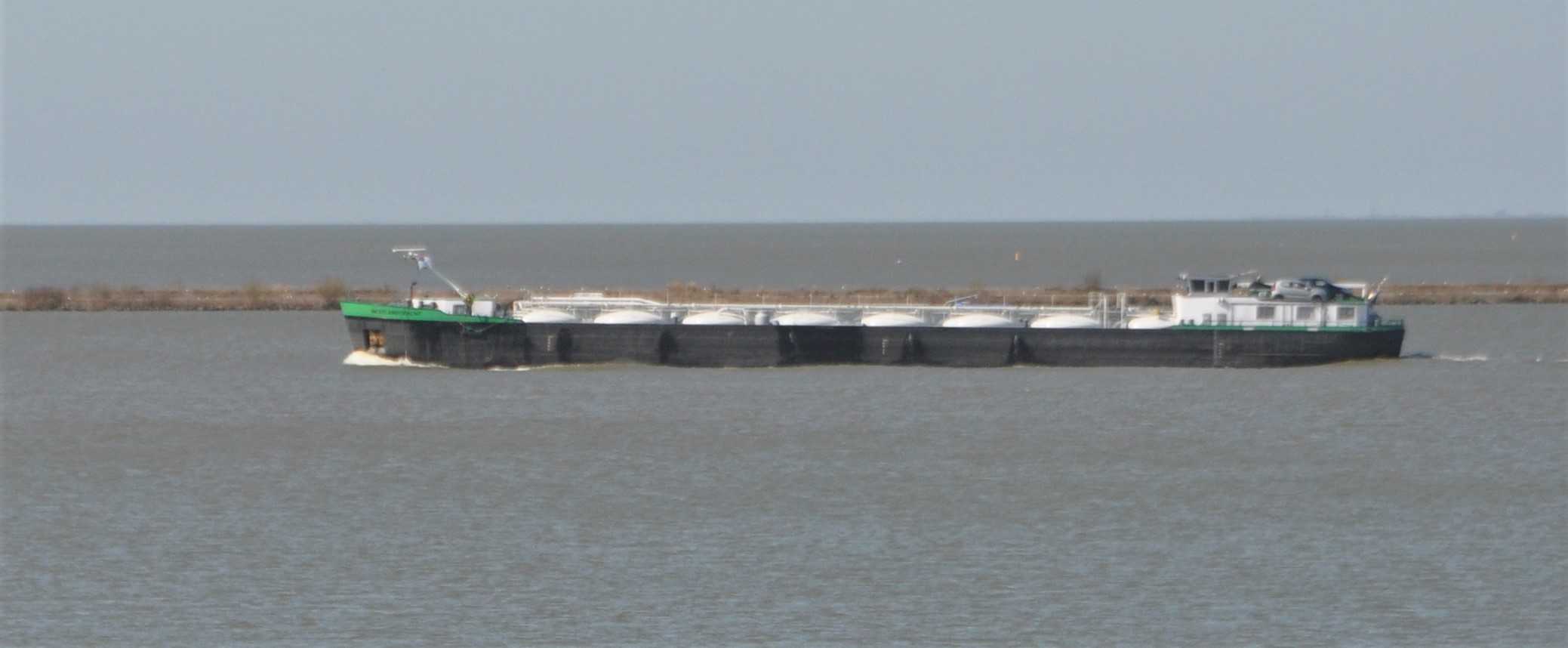In the image, a long, basic ship dominates the midsection, occupying approximately 75% of the horizontal space. The ship features a black bottom accented by green around its top and a white fence outlining its structure. Onboard, the vessel carries large, flat, white machinery along with some cars. Notably, a peculiar shadow effect gives the ship a segmented appearance. The water it sails on is murky, with hues of brown, grey, and dark green. Behind the ship is a natural-looking wall or barrier of green-brown land, likely intended to delineate parking boundaries for the ship. The backdrop features a calm, cloudy sky with a dull, grey tone, adding to the overall serene yet muted atmosphere.